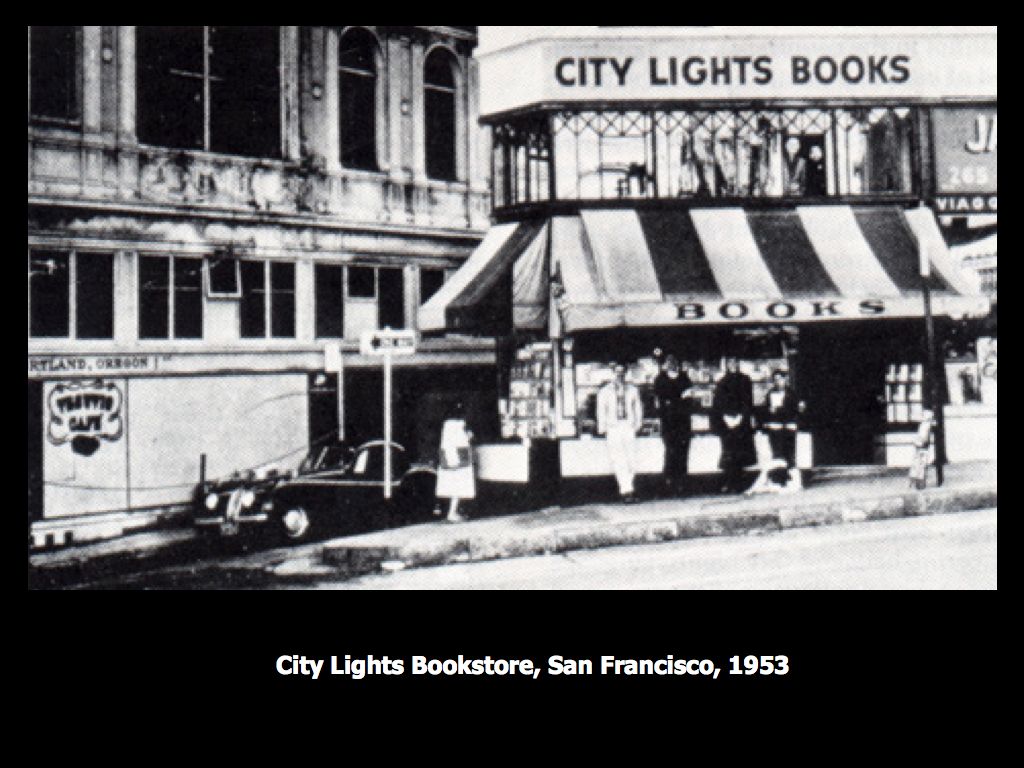The black and white photograph, a vintage snapshot from 1953, captures a city street scene in San Francisco. The image showcases two primary buildings. The leftmost building is a large, white structure adorned with large windows on the third story and smaller windows on the second story. The ground level features a blank white wall with a sign on the far left, though its text remains blurry and unreadable. A stylish, black vintage car is parked in front of this building. The centerpiece of the rightmost building is a sign with black lettering that reads "City Lights Books" across its façade. Below this sign lies a balcony, which stands above an awning that also bears the word "Books" in black letters. The awning itself has distinct black-and-white stripes. At street level, a book stand or newspaper stand can be seen with people milling around it; notably, a woman in a white dress engrossed in the selection of books. To the side, under the stand, several individuals are seen spectating, among them a person clad in a white suit contrasted by others in darker attire. The photograph's lower part has a caption, elegantly reading "City Lights Bookstore, San Francisco, 1953," marking the era and location of this timeless moment.